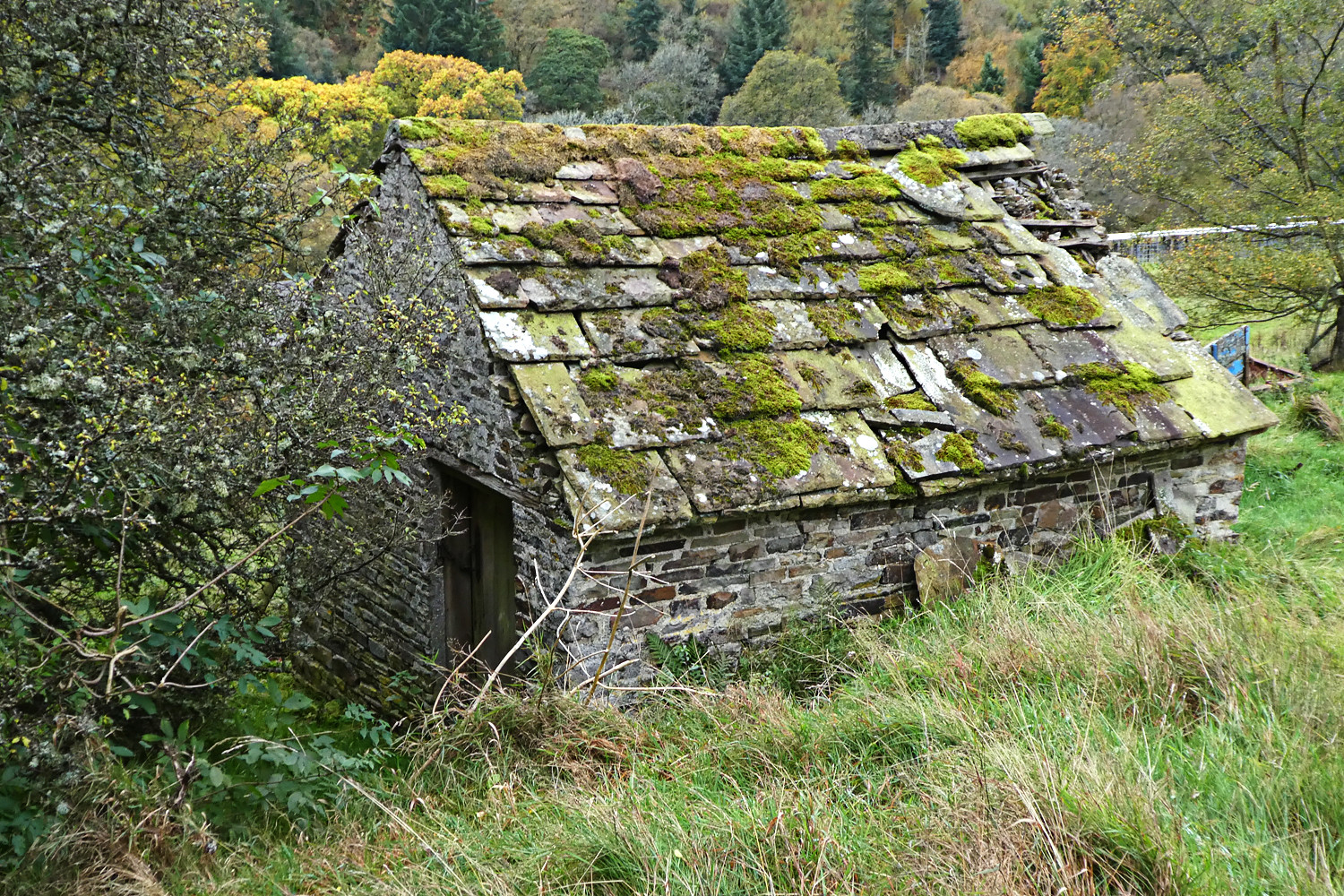An old, dilapidated stone shack, partially sunken into a dense, grassy area, is surrounded by thick weeds and numerous trees. The structure, with its grayish bricks, has a notably weathered appearance, featuring a small, closed wooden door on the left side of the building. The roof, covered in patches of green moss, has shingles that are damaged or missing on the right side. Tall grass, some browning and some green, stretches up to meet the walls, with earth accumulating more heavily on the nearer side of the structure. The background is filled with deciduous trees, some budding and others with larger leaves, creating a dense woodland atmosphere. Additionally, there appears to be a broken structure to the right of the shack, adding to the scene's overall sense of neglect and age.